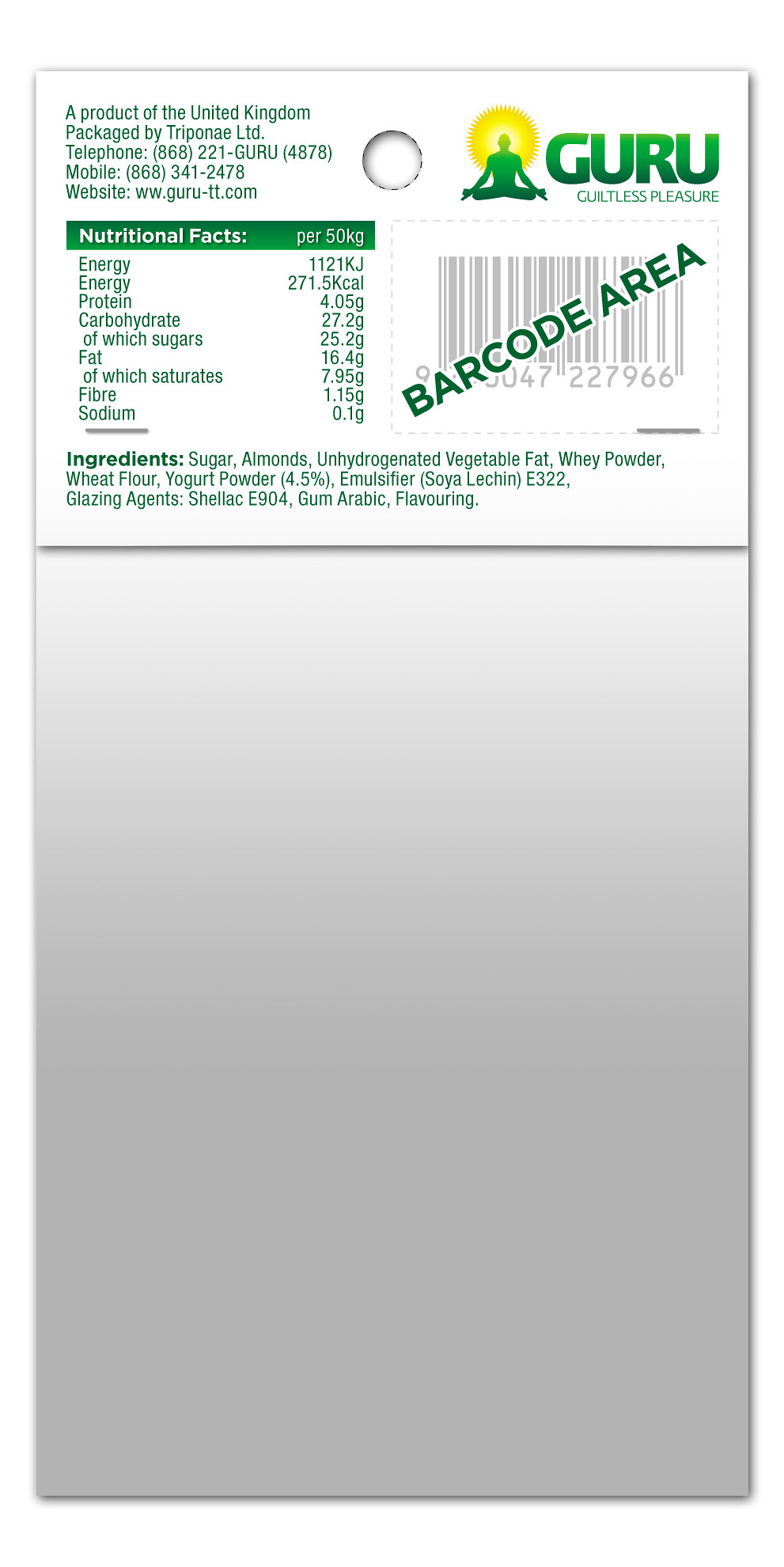This vertically-oriented rectangular image is predominantly divided into two distinct sections. The lower two-thirds of the image presents a plain, white-grayish background, while the top third features a product label rich in details.

The label, set against a pristine white backdrop, integrates green and yellow elements. In the upper left corner, it reads: "A product of the United Kingdom. Packaged by TriPonay Limited. Telephone: 868-221-4878. Mobile: 868-341-2478."

Directly beneath this information, against a green backdrop with white text, the label provides "Nutritional Facts per 50 kgs." This section details the nutritional content, including energy, protein, carbohydrates, sugars, fat, fiber, and sodium. Following this nutritional summary, the ingredients are listed as sugar, almonds, and dehydrated vegetable fat.

On the upper right corner of the label, the company’s branding is prominently displayed. The name "Guru Guiltless Pleasure" is shown alongside a symbolic image – an outline of an individual in a yoga pose, silhouetted against a yellow sun.